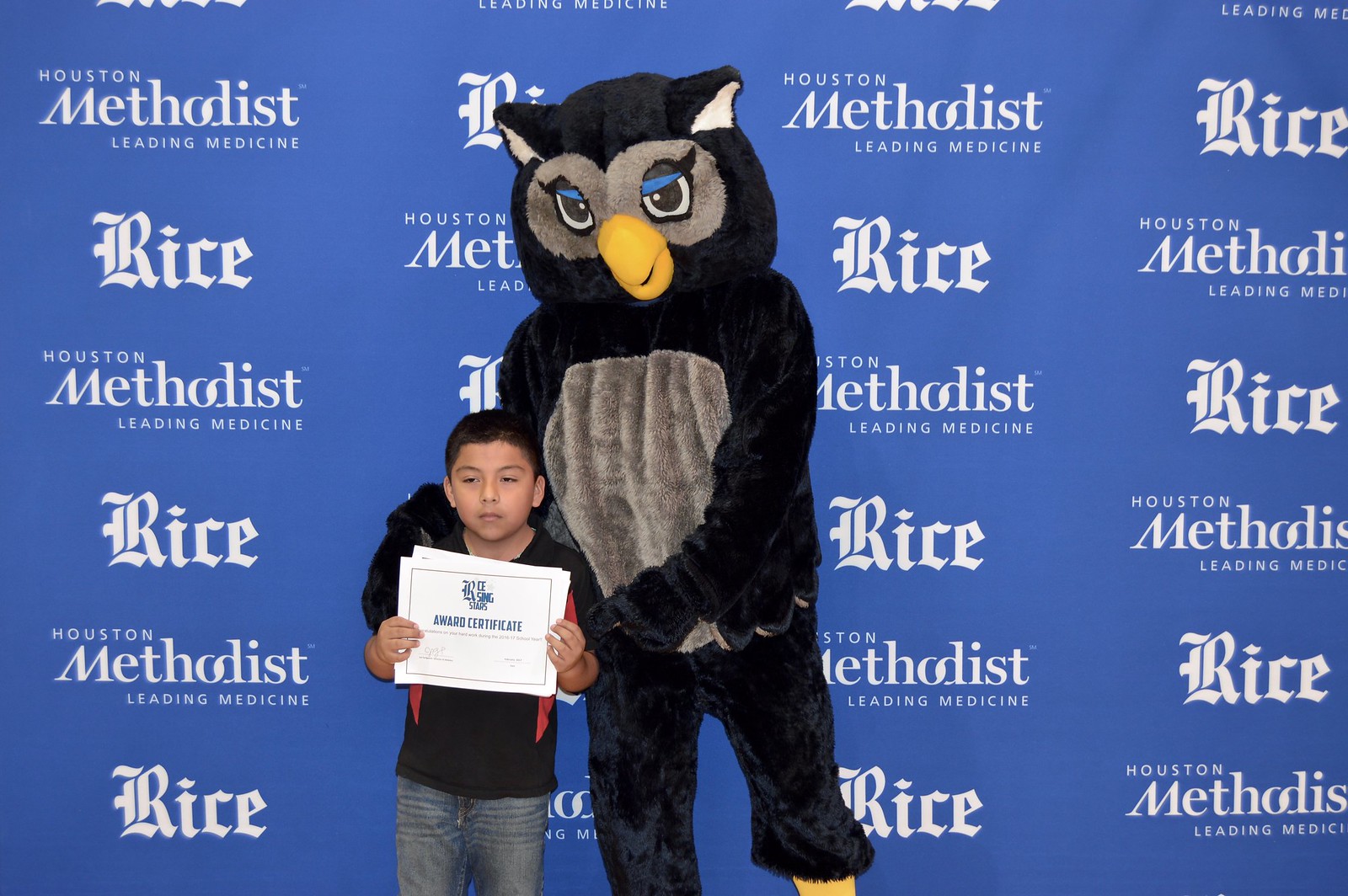A young boy, dressed in a black and red shirt with blue jeans, stands against a blue backdrop featuring a repetitive pattern of logos including "Houston Methodist Leading Medicine" and "Rice" emblazoned in thick gothic font. The boy, who appears somewhat disinterested or bored, is holding up an award certificate. Beside him is a person dressed in a black owl mascot suit with gray accents, including the belly and the area around the eyes, along with blue eyelashes and a yellow beak. The owl’s right hand rests on the boy's shoulder while the other hand supports the boy's arm, adding to the formal pose for the photograph.